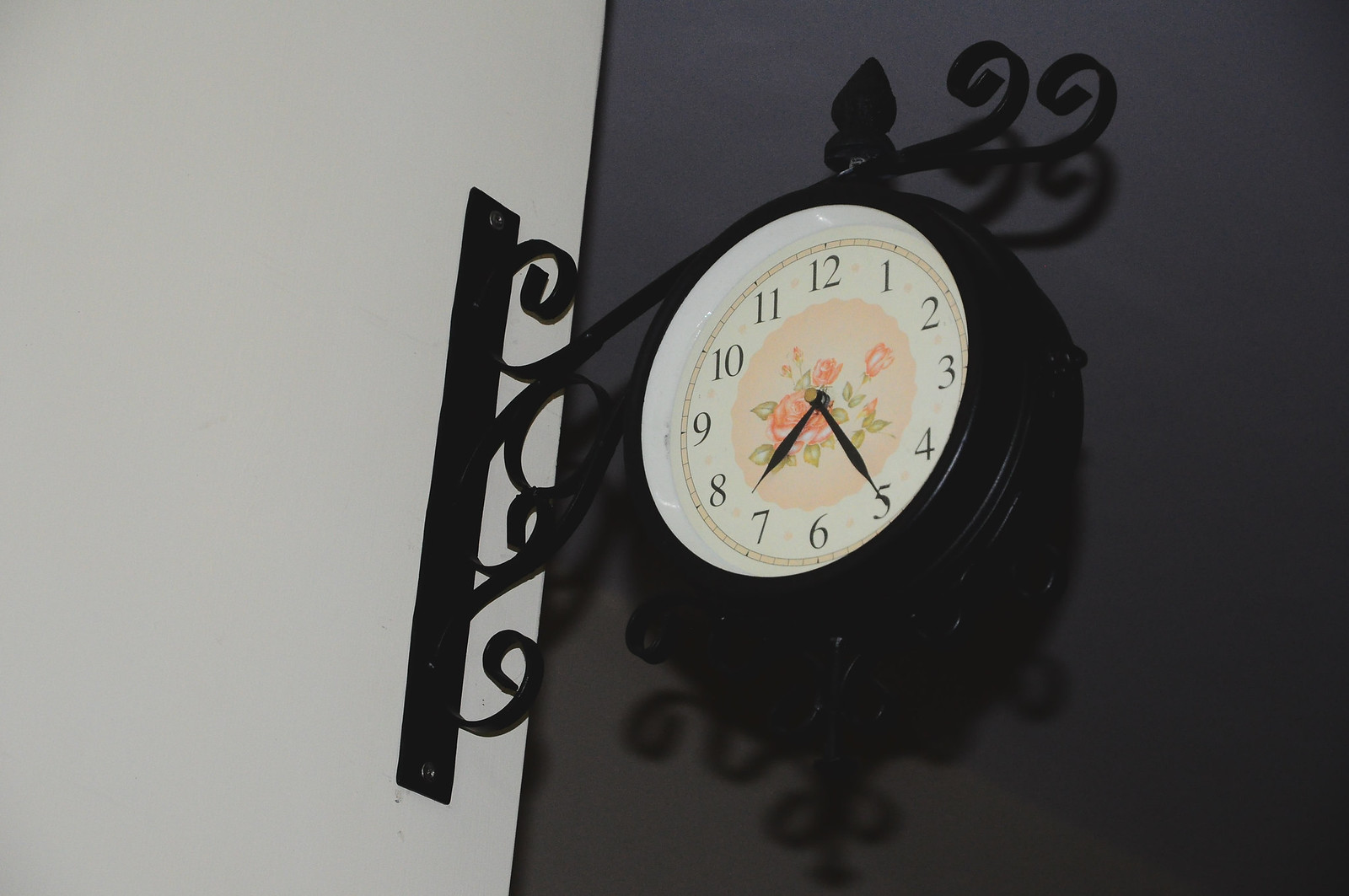The image showcases a round metal clock mounted on a white wall. The clock is attached to an ornate, black iron scrollwork that extends from a metal rod secured to the wall with screws at both the top and bottom. The clock features a white dial with a golden band circling the numbers, which are prominently displayed in black. At the center, a pink round area adorned with what seems to be a delicate arrangement of pink roses and green leaves adds a touch of elegance. The time displayed on the clock is 7:25.